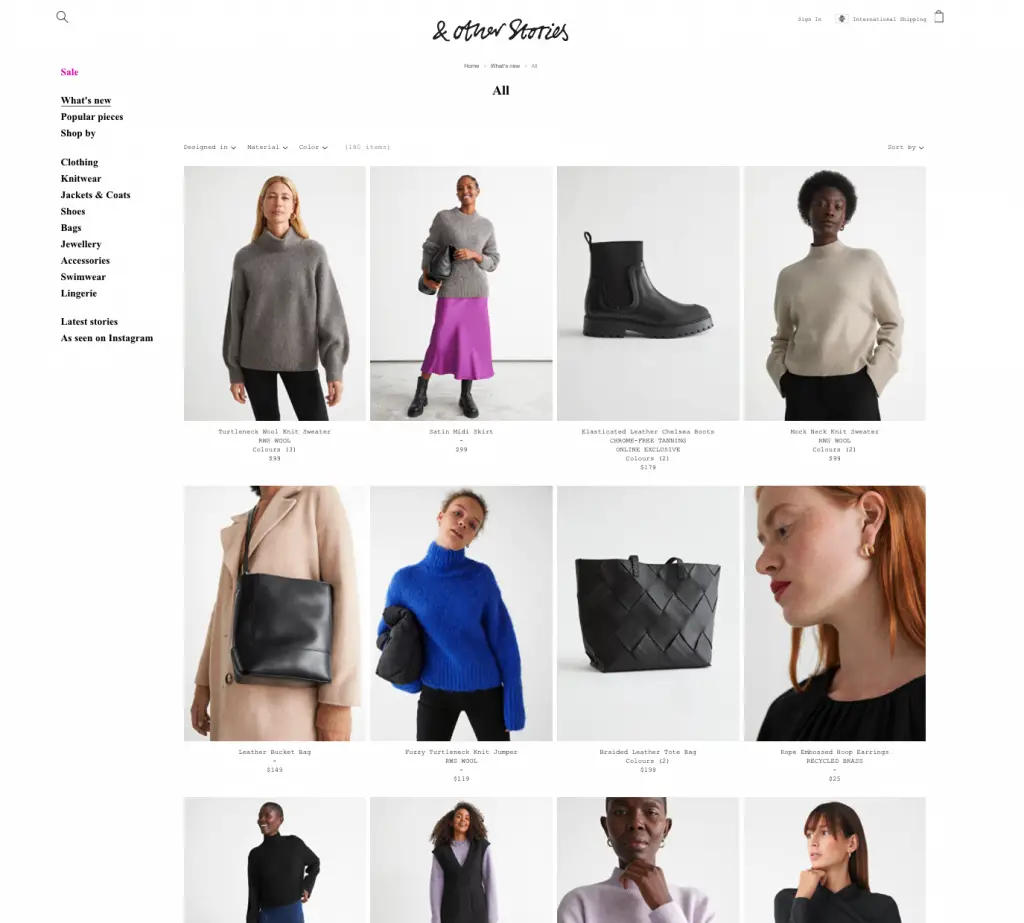A detailed and descriptive caption could be:

"This image captures a screenshot of a sophisticated website shopping page with a clean, white background. At the top left corner, there's a light gray magnifying glass icon representing the search function. Centralized at the top, in a stylish black handwritten font, is the text '& Other Stories,' showcasing the website's name. Adjacent to this, at the far right, 'Sign In' is displayed in light gray text, followed by a white box with a light gray outline that contains an indistinct dark gray icon. To the right of this box, 'International Shipping' is inscribed in light gray text, and further along to the right, a light gray shopping bag icon indicates the cart section.

Directly below the title, additional navigation links are placed centrally: 'Home' in dark gray text, followed by a light gray right arrow pointing towards 'What's New,' and another light gray right arrow pointing towards 'All.' Immersed below this navigation bar, the page emphasizes 'All,' inscribed in bold black serif text.

On the left, a vertical sidebar against the white background, initiates with 'Sale' in eye-catching pink text at the top. Following two line breaks, 'What's New' is underlined in black serif text, suggesting a highlighted option. Below, two lines read 'Popular Pieces' and 'Shop By' in the same black serif font, without underlines. Continuing downward, a list of categories separated by line breaks includes: 'Clothing,' 'Knitwear,' 'Jackets and Coats,' 'Shoes,' 'Bags,' 'Jewelry,' 'Accessories,' 'Swimwear,' and 'Lingerie,' each item written in black serif text, providing a clear and structured view of the website's offerings."